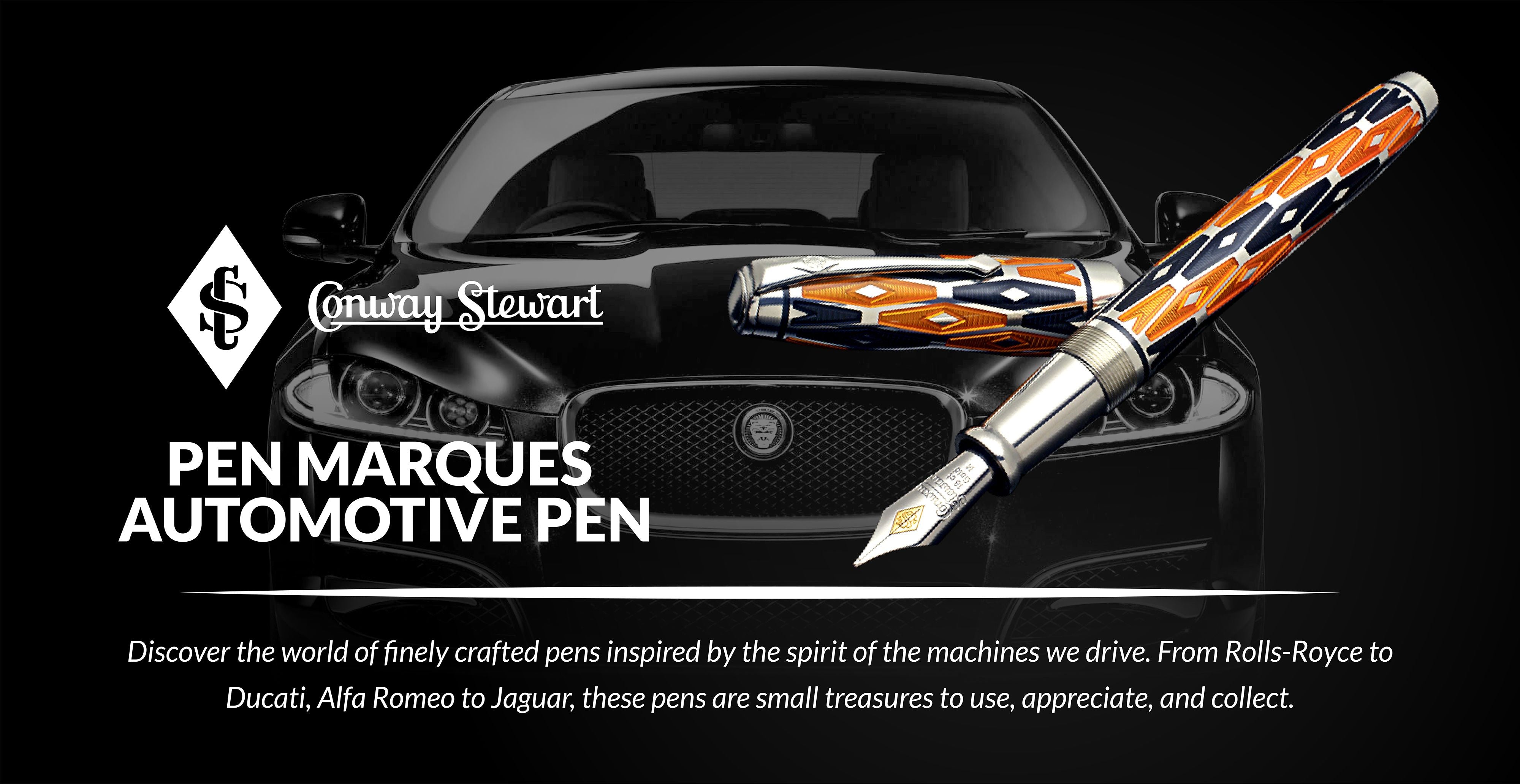This digital poster features the sleek front view of a glossy black sports car set against a black background. To the left, white text reads, "Conway Stewart Pen Marquis Automotive Pen." Adjacent to this text, there is an open pen rendered in silver, orange, and dark blue, with its matching cap displayed laterally in front of the car hood. The pen showcases a black and orange diamond pattern. At the bottom of the poster, white text declares, "Discover the world of finely crafted pens inspired by the spirit of the machines we drive. From Rolls-Royce to Ducati, Alfa Romeo to Jaguar, these pens are small treasures to use, appreciate, and collect." The poster showcases the luxury and design of both high-end automobiles and finely crafted writing instruments.